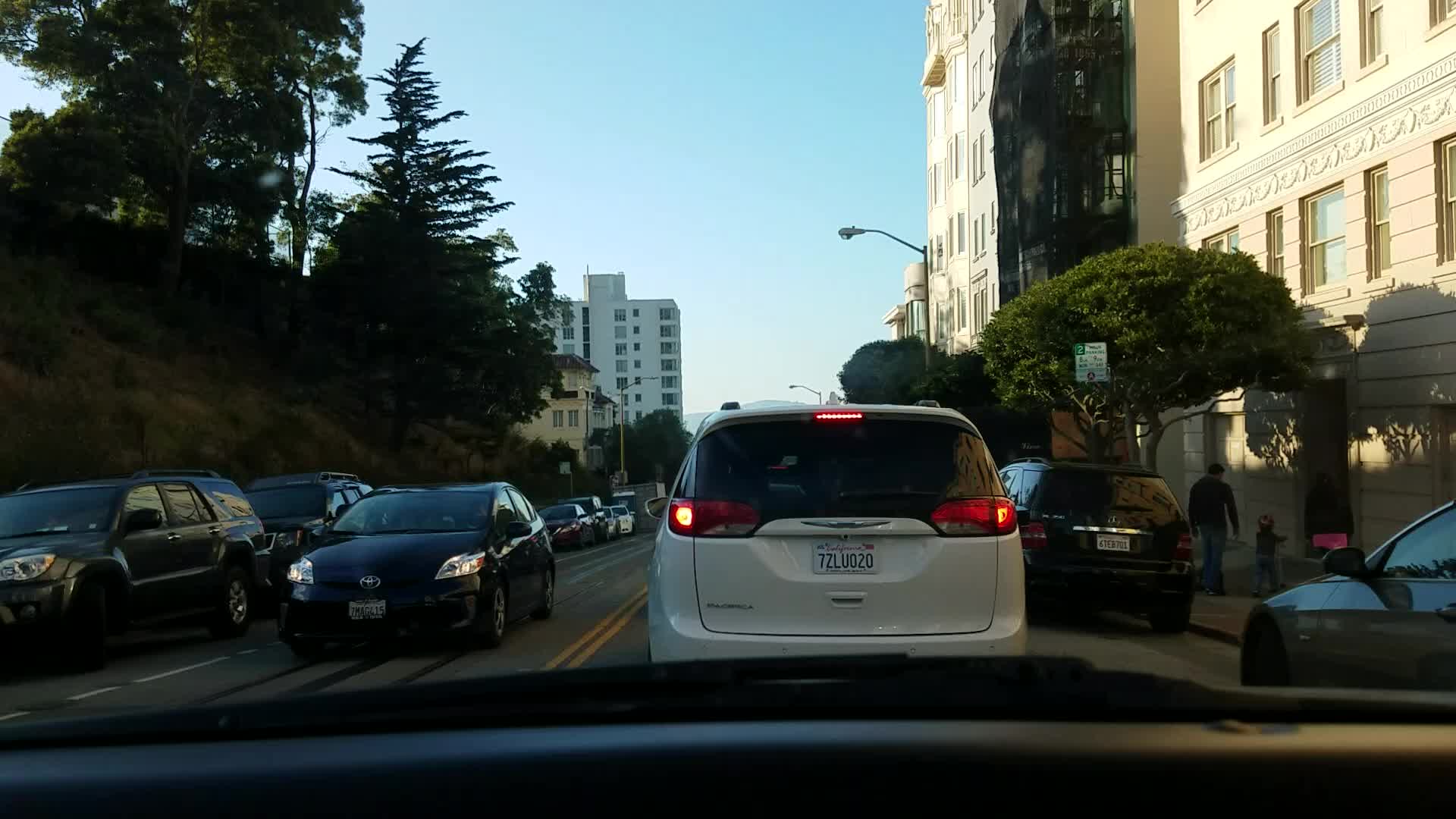This image captures a moment from inside a car traveling down a four-lane street, likely in an urban downtown area. Central to the scene is the back of a white van in the same lane as the photographer. To the right of the car, there are two additional lanes filled with various cars. To the left side, a grassy hill adorned with trees provides a touch of nature amidst the urban setting. On the right side, several beige buildings line the street, identifiable as part of the downtown landscape. A streetlight stands prominently while a man and a child are seen walking on the sidewalk, seemingly about to enter one of the buildings. A green and white parking sign is also visible, indicating nearby parking facilities. The overall picture paints a bustling city scene with a mix of vehicular traffic, pedestrians, and urban infrastructure.